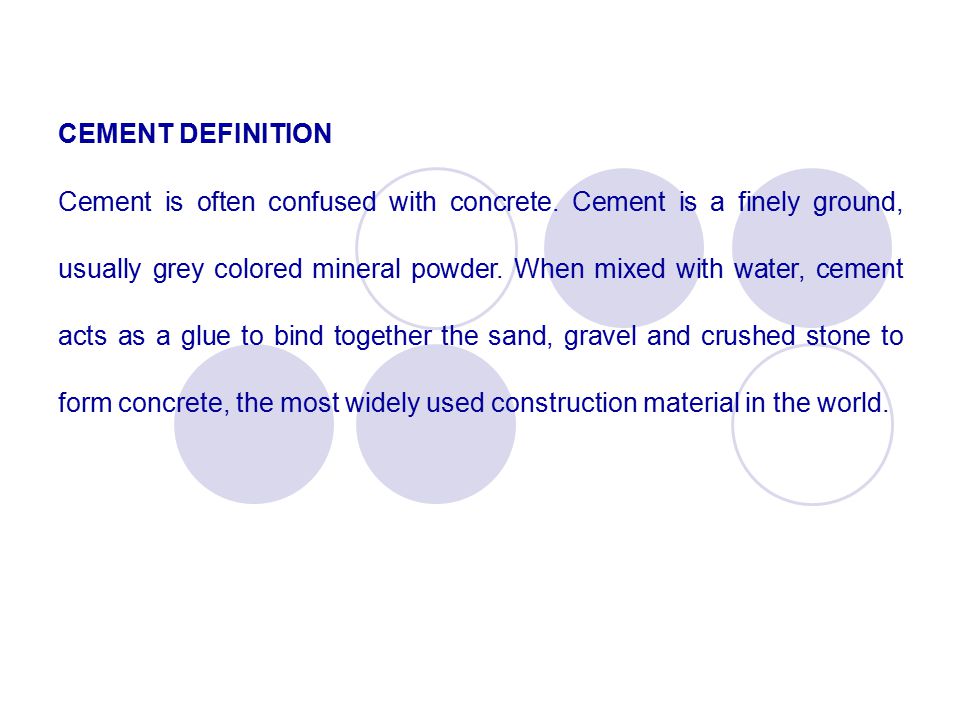The image features a detailed definition of cement, predominantly displayed in blue, bold, all-cap letters with a white background. Below the headline, the following text reads: "Cement is often confused with concrete. Cement is a finely ground, usually gray-colored mineral powder. When mixed with water, cement acts as a glue to bind together the sand, gravel, and crushed stone to form concrete, the most widely used construction material in the world." The background includes a total of six circles—four filled in with a light purple color and two unfilled white ones. These circles are scattered around the text; the first one is an unfilled circle, followed by two filled ones on the right side, then towards the bottom, there are two filled circles on the left and in the middle, and one unfilled circle on the right. These elements add a decorative touch, subtly highlighting the definition.